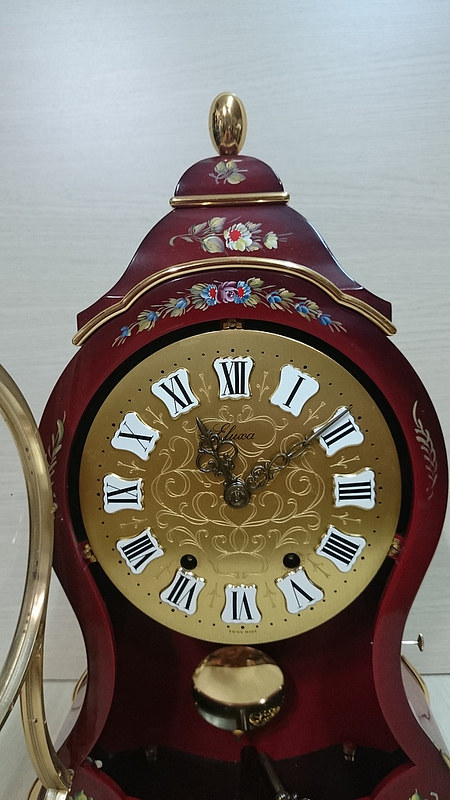The image features an antique, old-fashioned clock with a detailed and ornate design. The clock itself has a gold face with black Roman numerals and intricately designed hour and minute hands made of dark metal. The face also has pewter filigree etching, enhancing its elegance. The time displayed on the clock is approximately 11:09. This golden clock face is housed in a richly ornate, dark maroon casing that is adorned with painted flowers and a decorative gold knob at the top, resembling the top of a teapot or an urn. Beneath the clock face, a shiny golden pendulum swings back and forth. The clock casing has an open design, and the background of the image is white or slightly off-white. The entire piece exudes an antique charm, reminiscent of a bygone era, with fine craftsmanship visible in every detail.